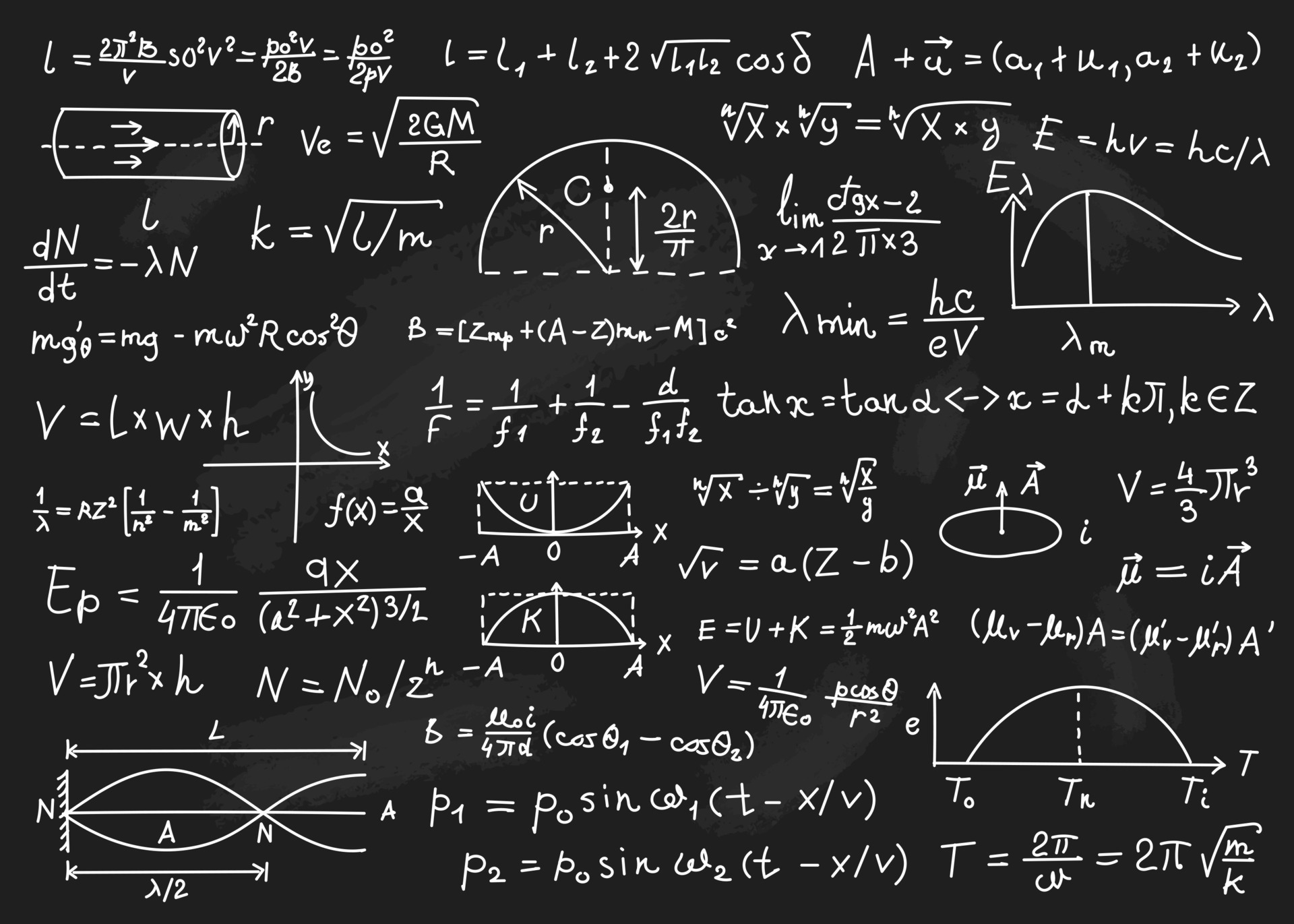This image is a highly detailed, digitally-created representation designed to mimic the appearance of a chalkboard. The black background, adorned with realistic-looking chalk smudges and fake erasure marks, adds to the illusion of an actual blackboard. The board is densely packed with an array of complex mathematical equations and formulas that span a variety of topics. These equations, which are written in mock handwriting with a white marker, cover the entire surface of the image, leaving hardly any empty space. Amidst the equations, there are nine distinct physical graphs, including line graphs and circular diagrams with directional arrows. Specific examples include the quadratic formula, the formula for velocity, a diagram illustrating the flow through a tube, and a graph depicting the relationship between energy and wavelength. The image also features various letters, numbers, and symbols, as well as a depiction of a cylinder with arrows pointing to the right. The overall effect is an intricate, AI-generated image that convincingly imitates a cluttered, chalkboard filled with mathematical content.